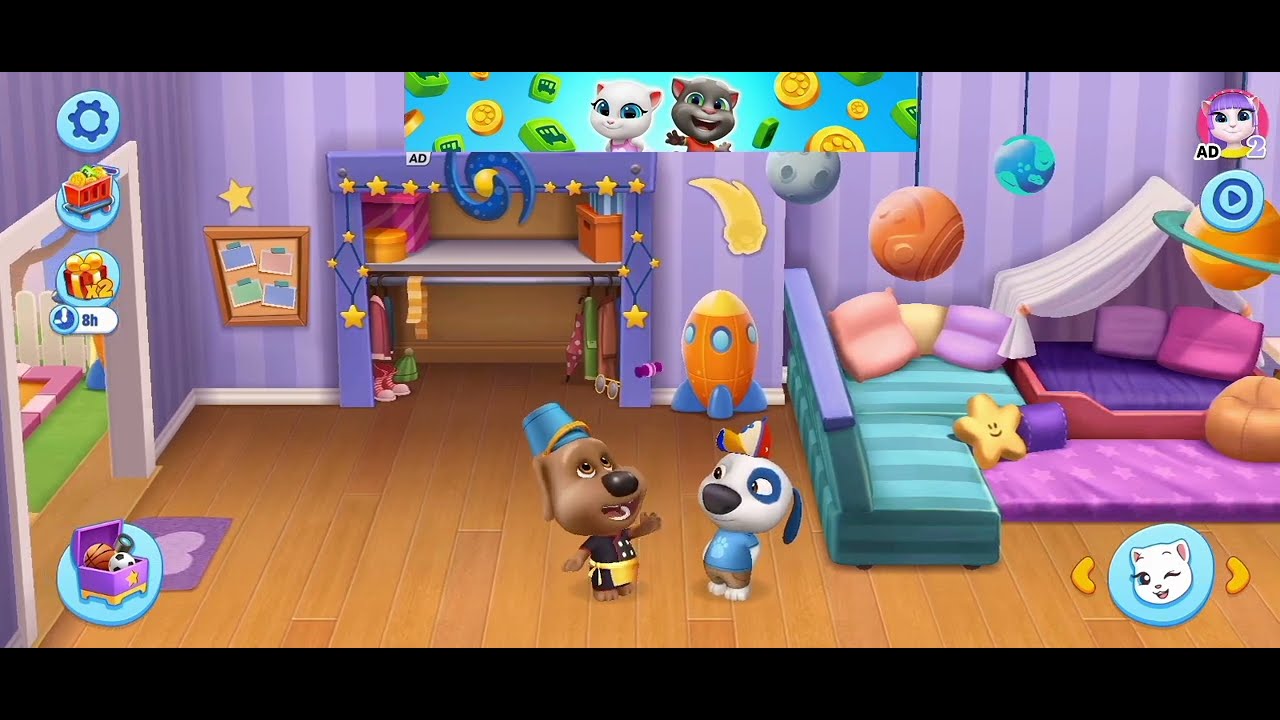The image appears to be a colorful, whimsical scene from a children's video game featuring a cartoon-like style. The setting is a vibrant bedroom with light purple and darker purple striped walls, wooden flooring, and numerous decorative elements. In the bottom center are two anthropomorphic dogs. The left dog is brown, wearing an apron and a fez-like hat, while the right dog is white with a blue circle around his eye, dressed in a blue t-shirt and brown pants. 

The room is adorned with various playful objects: a bed with a canopy to the right, a couch with pillows, and a small rug in front of the bed. There is a creatively made fort or tent with white cloth, suggesting a cozy nook for pets. In the background, stars and planets hang from the ceiling, adding to the dreamy atmosphere. There's also a globe and hanging objects including a basketball and replicas of the Earth.

Behind the white dog, a roller skate, rocket, and other toys are scattered around. Coins with paw prints and green boxes float in the background, enhancing the sense of whimsy. A photograph or perhaps a window reveals two smiling cats, one white and one gray, with big blue eyes. To the left, a doorway shows a glimpse of a white picket fence and a tree outside. The room also features a small walk-in closet with a clothing rack and hat boxes. Lastly, a little treasure box on the left contains two balls. The overall scene is packed with engaging, colorful details that capture a child's wonder and imagination.